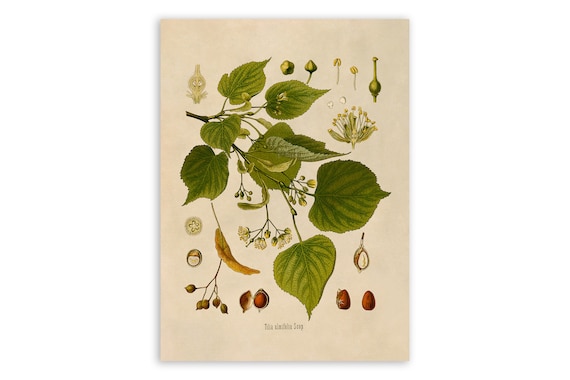This image is a detailed, somewhat faded drawing on a light brownish-white background, resembling an illustration from an old botanical textbook. The focal point is a close-up of a sprig featuring nine lush green leaves with tapered shapes and prominent veins. The leaves are nourished by a central vein with smaller veins branching off. Among these green leaves are several small flowers, either light white or yellow, with visible pistons and stamens, suggesting they are in bloom. Additionally, the illustration includes various other plant elements such as buds, seeds, nuts (some of which appear cut open), and smaller branches with flowers in shades of yellow, green, and brown. In the upper right corner, there are sprigs with unopened flowers or buds. The bottom of the image contains a Latin script in a faded gray color, which is largely unreadable. Overall, the composition is detailed but not hyper-realistic, capturing an array of botanical features with a scientific yet artistic touch.